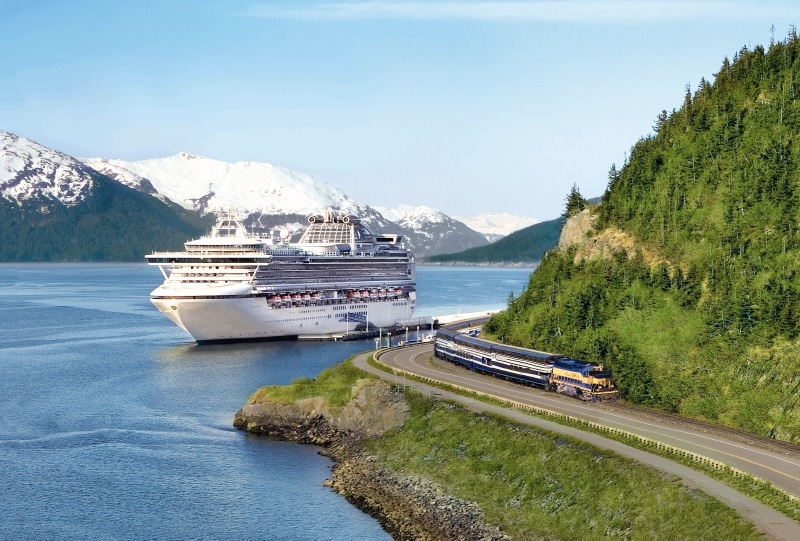The image captures a stunning mountainous landscape, likely in Alaska, with clear blue skies overhead. Dominating the scene on the left is a vast, serene lake with deep blue waters, where a large, white multi-deck cruise ship is either docked or moving slightly towards the bottom left. On the right side, a yellow and blue train runs parallel to a paved road, weaving its way along the base of a forested mountain. This mountain, covered in lush green trees, transitions to snow-capped peaks as it moves further back in the frame. Opposite this, across the lake, lie more snow-covered mountains that complete the picturesque backdrop. The color palette involves light blue skies, darker blue waters, greens of the hills and trees, white for the snow and the cruise ship, and the vibrant yellow and blue train, creating a visually rich and busy scene.